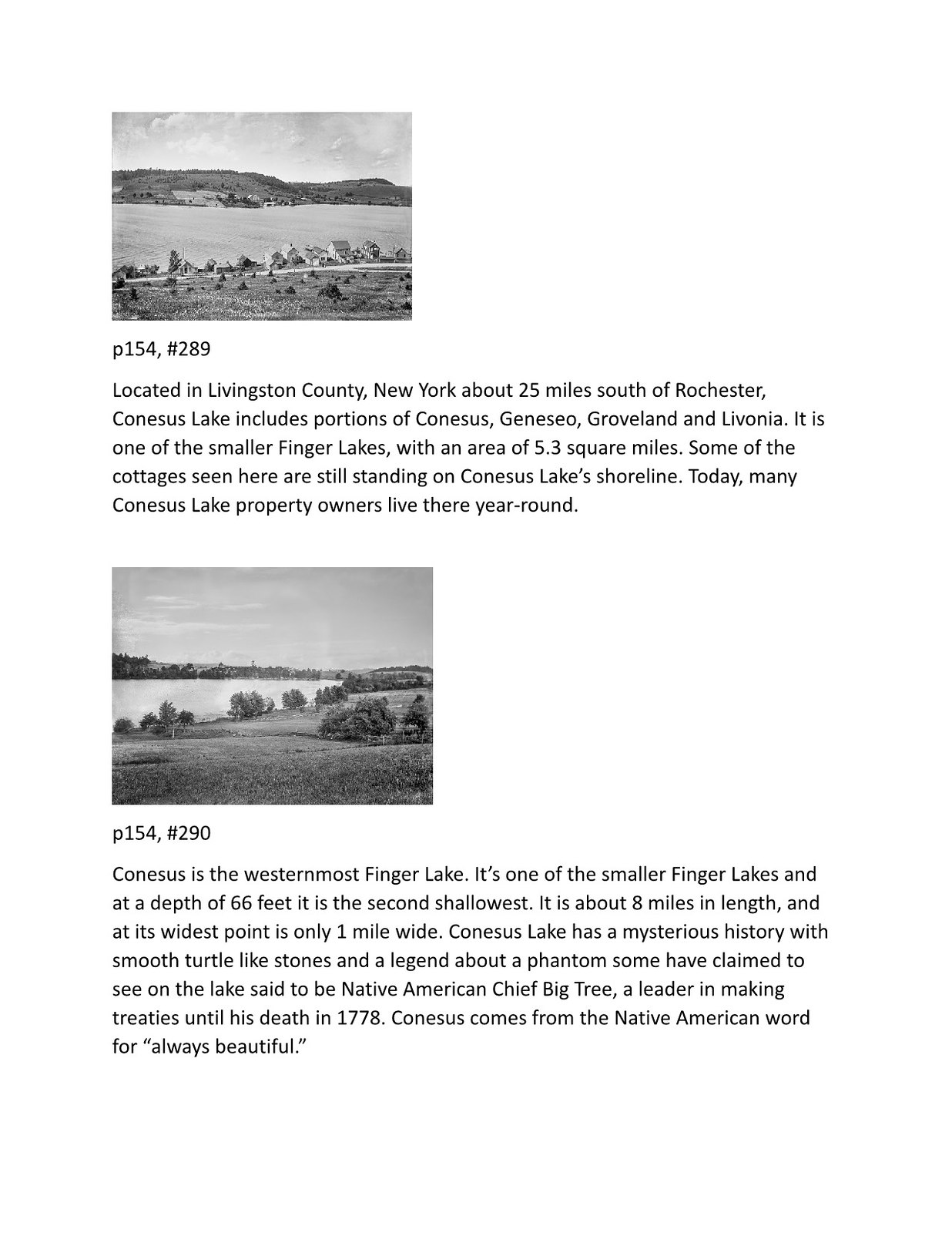The image appears to be a scanned black-and-white page, possibly from a textbook, featuring two photographs and corresponding text blocks. The top photograph shows a row of cottages interspersed with sheds or barns in front of a large open field with rolling hills and a gravel road. This image, marked as page 154, number 289, is located in Livingston County, New York, approximately 25 miles south of Rochester. It depicts the Kinesis Lake area, which encompasses parts of Kinesis, Geneseo, Groveland, and Livonia. Kinesis Lake, one of the smaller Finger Lakes at 5.3 square miles, has some cottages still standing on its shoreline where many property owners now reside year-round.

The bottom photograph, also labeled as page 154, number 290, captures a forested hillside next to a large open lake with trees and buildings on its far side. This lake, named Kinesis, is noted for being the westernmost of the Finger Lakes and is among the smaller lakes, measuring about eight miles in length and one mile at its widest point. Kinesis Lake is the second shallowest Finger Lake with a depth of 66 feet. Known for its mysterious smooth turtle-like stones, the lake carries a legend of a phantom, said to be the Native American Chief Big Tree, who passed away in 1778. The name Kinesis is derived from a Native American word meaning "always beautiful."